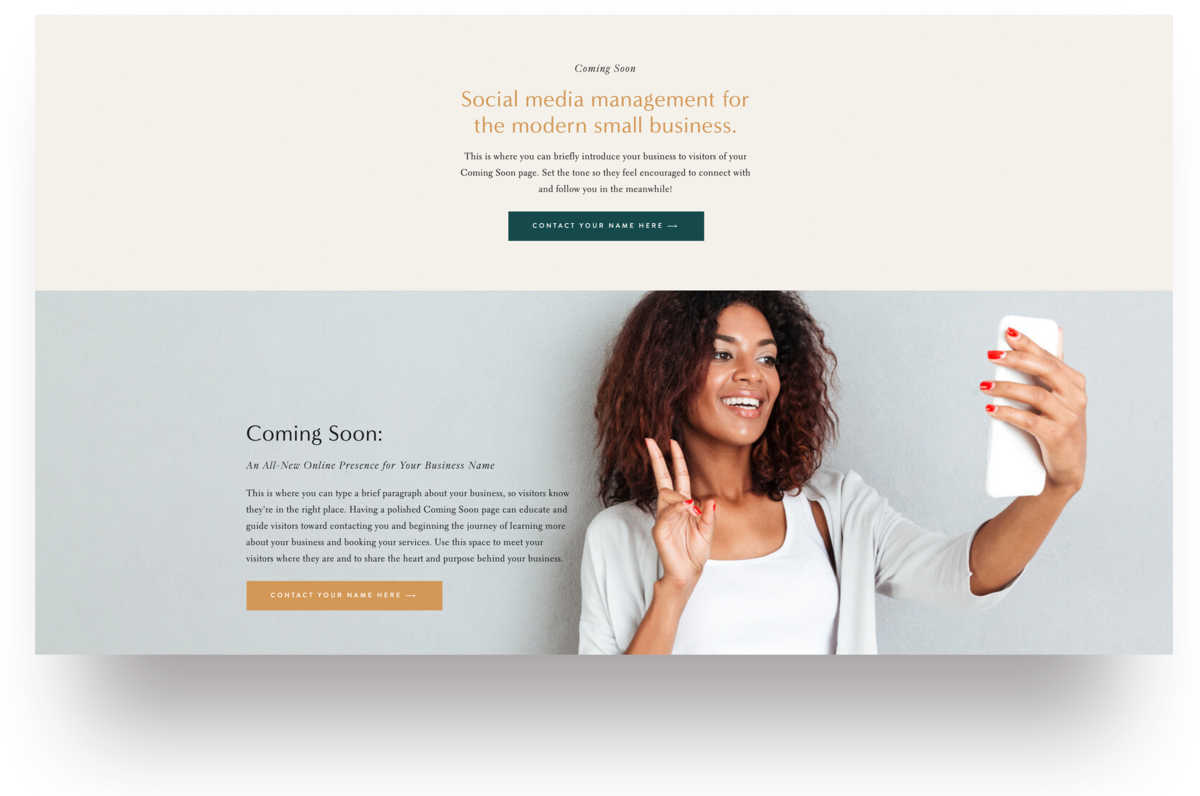The image is a screenshot of an announcement for an upcoming service, featuring the following elements:

1. **Banner Text**:
   - At the top, the banner displays the phrase "Coming Soon" in clear, bold letters.
   - Below it, in brown text, there's a headline that reads, "Social Media Management for the Modern Small Business."

2. **Description Section**:
   - Under the headline, there's a block of very small, pixelated text, making it hard to decipher. It appears to provide a brief introduction to the service, possibly mentioning something about launching a business, but the blurry print renders it largely unreadable.

3. **Call to Action Buttons**:
   - Directly beneath the blurry text, a green button seems to prompt some action, likely saying "Contact Us" or a similar call to engage.
   - Another call-to-action button in orange, located at the bottom left of the image, suggests connecting further, but the exact wording remains indiscernible due to pixelation.

4. **Image of a Person**:
   - Prominently featured is a picture of a brown-skinned woman making a peace sign and taking a selfie.
   - Her shoulder-length hair frames her face, and she is dressed in a white blouse with medium-length sleeves layered over a sleeveless tank top.

5. **Additional Text**:
   - Near the bottom, there's another small, blurry text area that appears to mention an "online franchise for your American name" or something similar, but the precise details are obscured due to the poor image quality.

The overall layout is modern, targeting small businesses interested in social media management solutions, and it includes visual elements aimed at engaging the audience despite some challenges with text clarity.